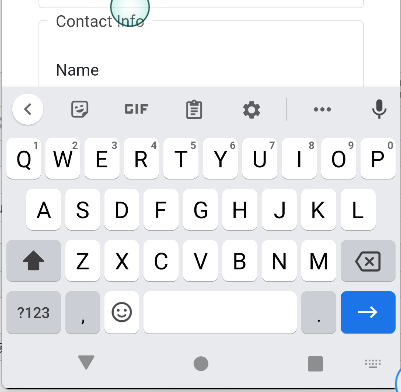This image captures a screenshot of a cell phone interface, showcasing a partially displayed keyboard along with a small section of a webpage. The keyboard, primarily in shades of gray, white, and black, features a prominent blue square with a white forward arrow in the bottom right-hand corner.

On the main screen, the keyboard is actively popped up, obscuring most of the page behind it. The visible portion of the page reveals a section titled "Contact Info" in bold black letters, followed by the label "Name," also in bold. Above the phrase "Contact Info" is a partially visible, semi-translucent bluish-green dot, positioned towards the top of the screen and partly cut off.

The background beneath the keyboard is notably gray, while the top of the screen includes navigation elements. On the left side, there's a white icon featuring a black back arrow. Adjacent to it is a square icon indicating stickers, a bold "GIF" label, a clipboard icon, and a gray gear icon symbolizing settings. A vertical gray line separates these elements from three horizontal black dots and a black microphone icon positioned further to the right.

The entire image is framed by light gray borders on the left, right, and bottom edges, contributing to the overall structured appearance of the screenshot.